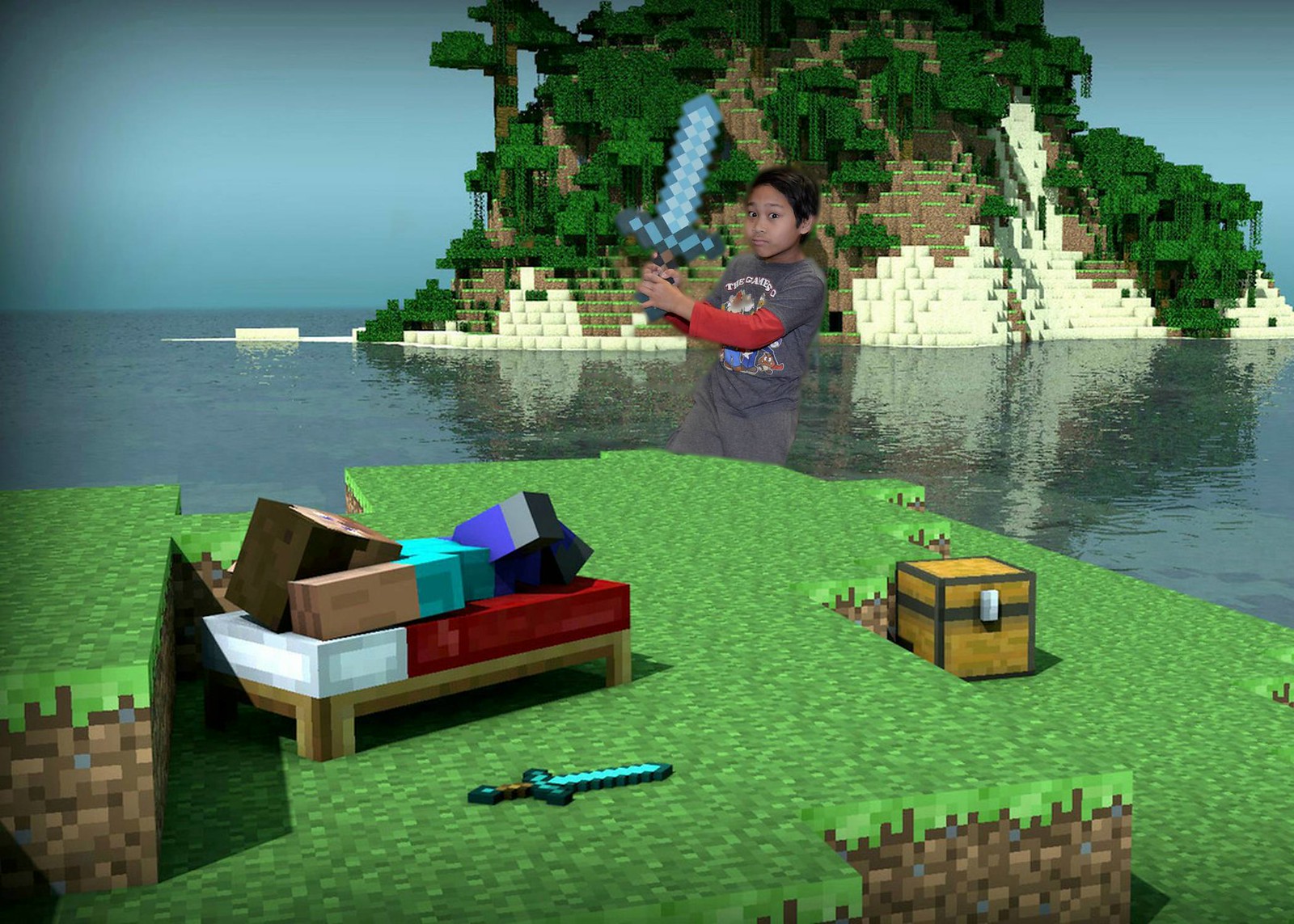The image is a digital collage blending an actual photograph with a scene from the video game Minecraft. The central focus is a young Southeast Asian boy with black hair, wearing a gray t-shirt layered over a red long-sleeve shirt. He stands upright, facing left, making a fierce expression, poised as if about to swing a pixelated Minecraft diamond sword that he holds in both hands. The Minecraft setting features the characteristic blocky landscape, with green grass blocks in the foreground and a square treasure chest with gray trim. A Minecraft bed with a character laying on it, a sword beside him, is also visible. In the background, Minecraft water stretches out to an island composed of dirt, sand, and blocky trees. This conceptual art piece effectively merges the real and virtual worlds, capturing the imaginative essence of Minecraft.